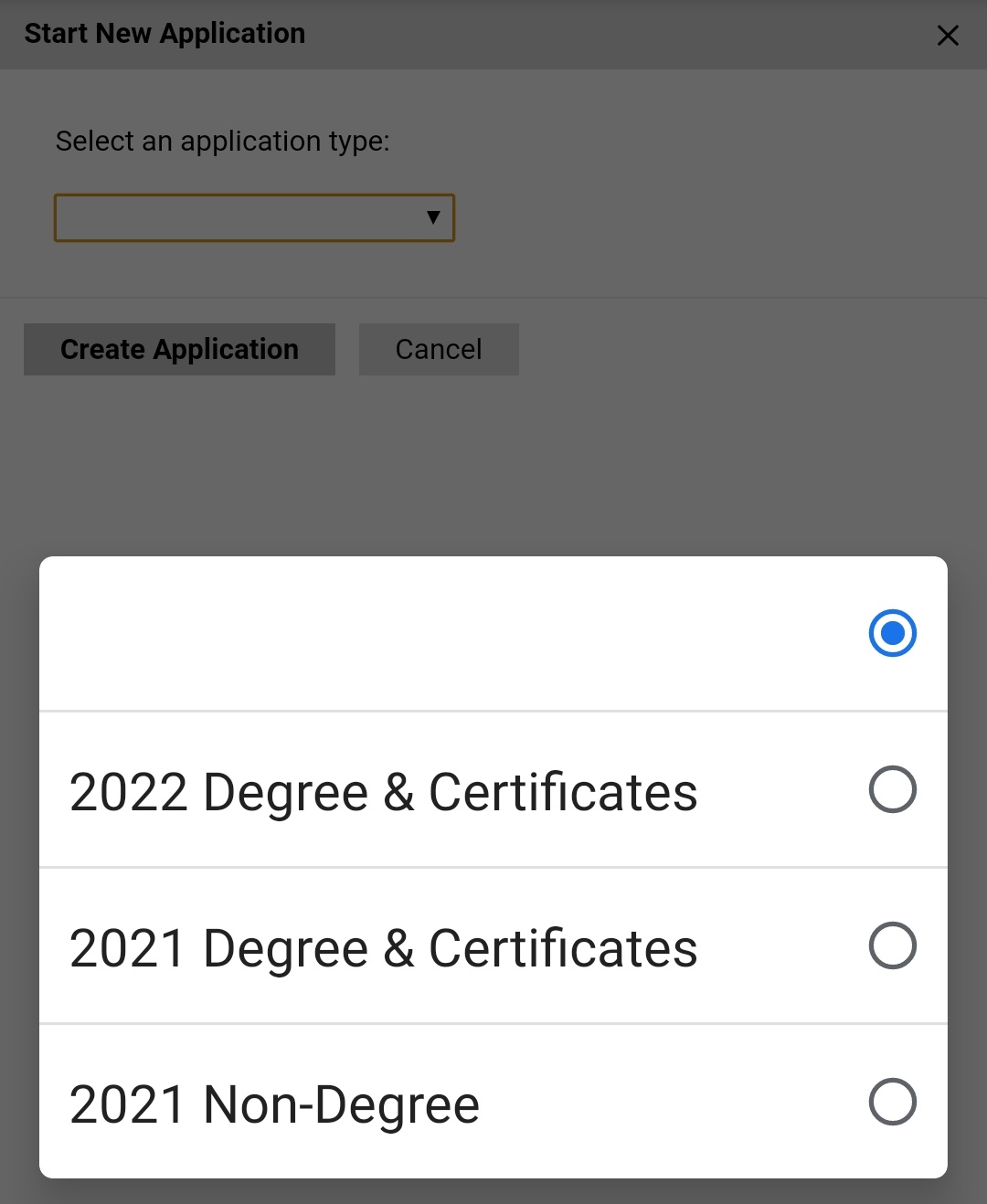A screenshot displays the interface of a mobile app or website. At the bottom of the screen, a white pop-up menu is visible, featuring four selectable rows each with a corresponding dot on the right to indicate selection status. The top row is marked by a blue-filled circle but has no text. The subsequent rows list options: "2022 Degrees and Certificates," "2021 Degrees and Certificates," and "2021 Non-Degree," all shown with blank circles. The backdrop of the image is gray, partly obscured by the bright pop-up section. The top left corner displays the text "Start New Application," while the top right corner features a clickable "X" for closing. Below this, a section bordered in orange prompts users to "Select an Application Type" via a drop-down menu. Bold black text reads "Create Application" with a gray "Cancel" button beside it.